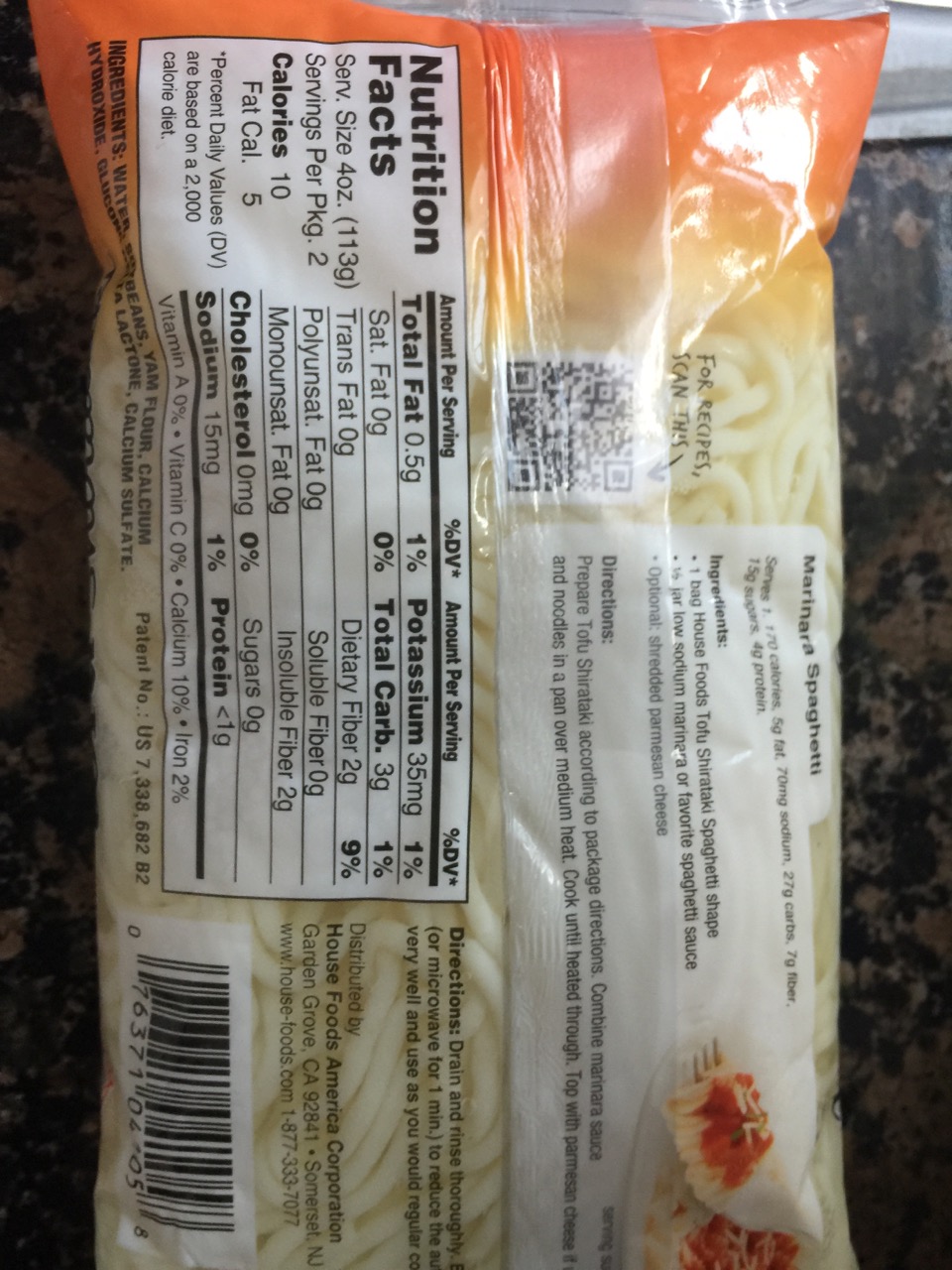A vertically-oriented color photograph depicts a bag of pasta noodles standing upright on an edge of a dark gray granite or marble countertop, characterized by various shades of brown and black dots. The image captures the bag tilted 90 degrees to the right, cropping off the top and bottom. The clear, shiny plastic packaging transitions from orange at the top to yellowish-orange, revealing slimy yellow noodles inside. On the lower left corner of the package, a white rectangular box displays nutrition facts, highlighting the item's potassium, carbohydrate, and fiber content. Adjacent to this is a black UPC barcode. Towards the lower right quadrant, a recipe for marinara spaghetti is visible, accompanying an image of noodles in sauce. Small black text lists the ingredients and distributor details, and the light source, possibly a flash, reflects off the bag, emphasizing its glossy surface. In the upper right corner of the image, part of a stainless steel kitchen sink can be seen.